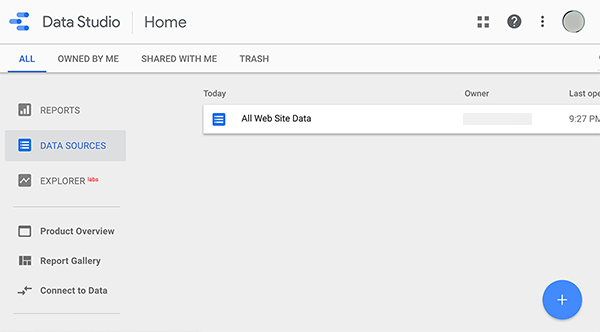The image showcases a screenshot of a computer screen displaying the Google Data Studio interface. In the top left corner of the screen, "Data Studio" is prominently displayed next to a "Home" button. On the top right, there is a blue circle with a white question mark inside it, signifying a help or support icon. Further to the right, in the extreme corner, there is a circle with a gray background, possibly representing the user profile or settings menu.

Beneath these elements, there's a navigation tab where "All" is highlighted in blue and underlined, indicating the current selection. Next to it are tabs labeled "Owned by Me," "Shared with Me," and "Trash." 

On the left sidebar, there are several navigation options. At the top is an icon resembling a square with three horizontal lines, labeled "Reports." Below it is another square with horizontal lines, highlighted in blue, indicating the "Data Sources" section. Beneath this, there is an icon with a zigzag line labeled "Explorer." Following this is an icon resembling a folder titled "Product Overview." Below, there is an icon of a gallery, labeled "Report Gallery." 

Further down, there are arrows pointing left and right next to the text "Connect to Data." To the right of the sidebar, the word "Today" is visible. Underneath, there is a blue square with horizontal lines labeled "All Website Data." The word "Owner" is displayed next to a text field that is obscured or redacted, making it unreadable. Adjacent to this, the text "Last Ope" is cut off by the edge of the page, with a timestamp reading "9:27 PM."

In the bottom right corner of the screen, there is a noticeable blue circle with a white plus sign in the middle, likely used to add new reports or data sources.